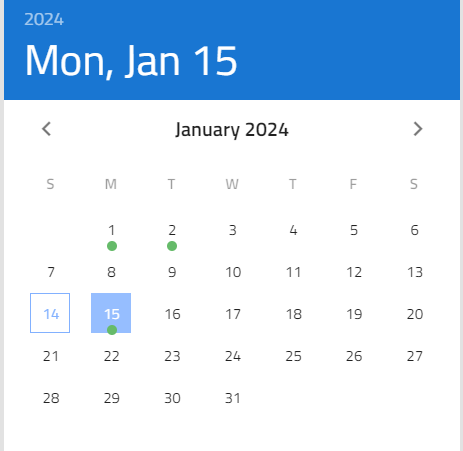This is a detailed screenshot of a calendar for January 2024. The calendar occupies a vertical rectangle. At the top of this rectangle, there is a horizontal blue bar. In the top left corner of the bar, the year "2024" is displayed in light blue text. Directly below, in larger white letters, the date "Mon, Jan 15" is prominently shown.

Below the blue bar is the main body of the calendar. On the top left of the calendar, there is a left-facing arrow, and in the center, the month "January 2024" is displayed in black text. To the right of this title, there is a right-facing gray arrow.

Beneath the title of the month, the days of the week are indicated by their initials: "S M T W T F S". The dates of the month follow beneath these initials, with the days arranged in a grid format. 

The first day of January 2024, a Monday, is placed under the "M". This date, as well as January 2nd, has a green dot underneath it. The dates continue sequentially across the row: 3, 4, 5, and 6.

On the next row, starting from Sunday, January 7th, the dates are displayed in gray. The progression of days continues, with January 8th being a Monday, January 9th a Tuesday, January 10th a Wednesday, January 11th a Thursday, January 12th a Friday, and January 13th a Saturday.

Highlighted within the calendar is a blue box containing the number 14 in white, indicating Sunday, January 14th. To the right of this, Monday, January 15th, also appears in a blue highlighted box with the number "15" in white and a green circle at the bottom of the box.

The dates continue to the end of January, with the month ending on Wednesday, January 31st.